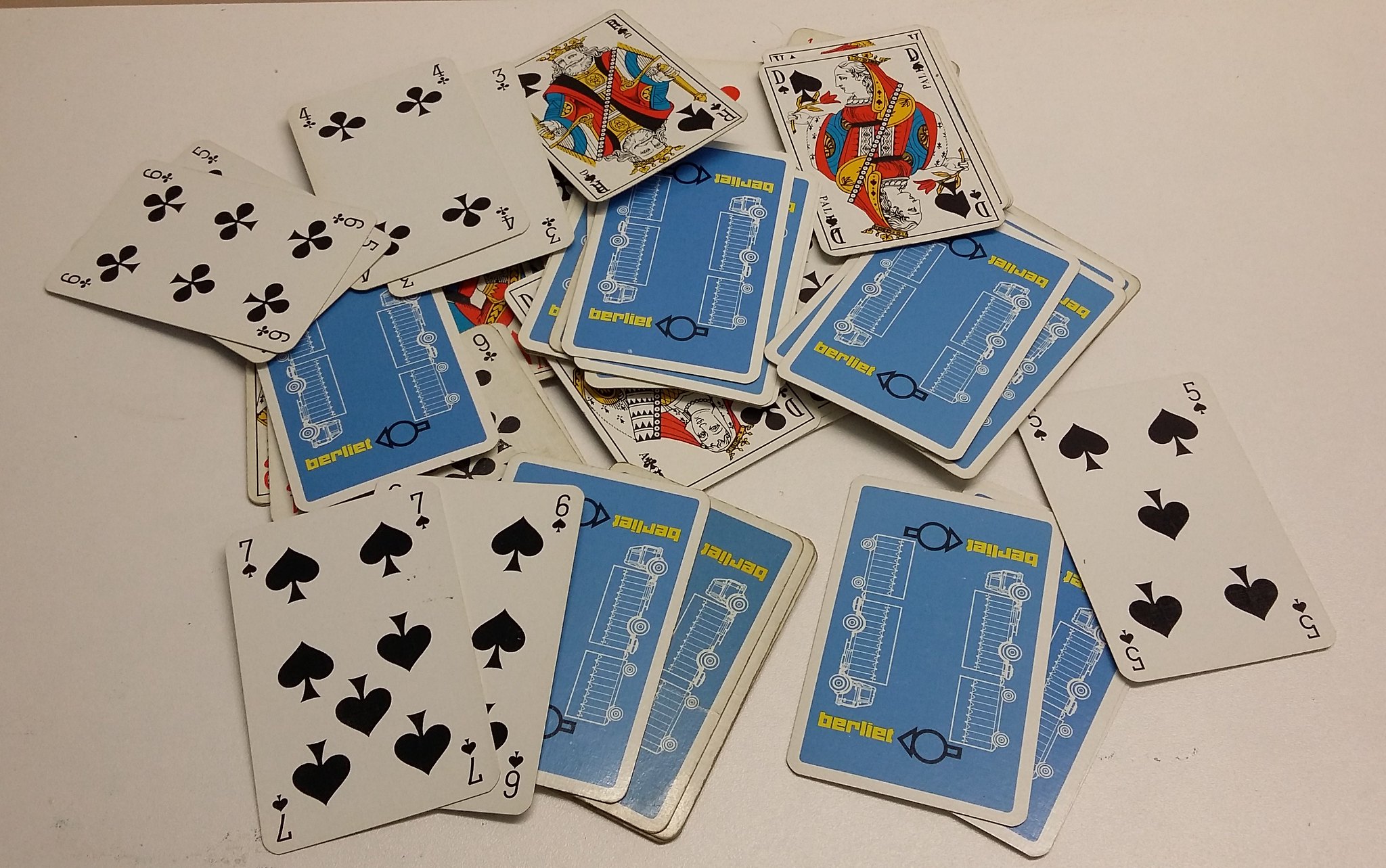The photograph features a white surface as the background, on which five distinct piles of playing cards are arranged in various positions. The top left pile consists of several cards, all face down. Moving to the middle top pile, it also contains face-down cards with the top card showing a King of Spades. 

The top right pile is more chaotic, displaying a mix of face-up and face-down cards, specifically showing the Six of Clubs, the Three of Spades, and the Four of Clubs. The backs of the cards are blue with some yellow writing and an illustration of a double-mat truck going both upward and downward on the card. 

Transitioning to the bottom half of the image, the bottom right pile includes three cards, with two face down and one face up revealing a Five of Spades. Lastly, the bottom left pile is composed of several face-down cards, with the top one shifted to the left. On top of these, the Six of Spades and the Seven of Spades are distinctly visible.